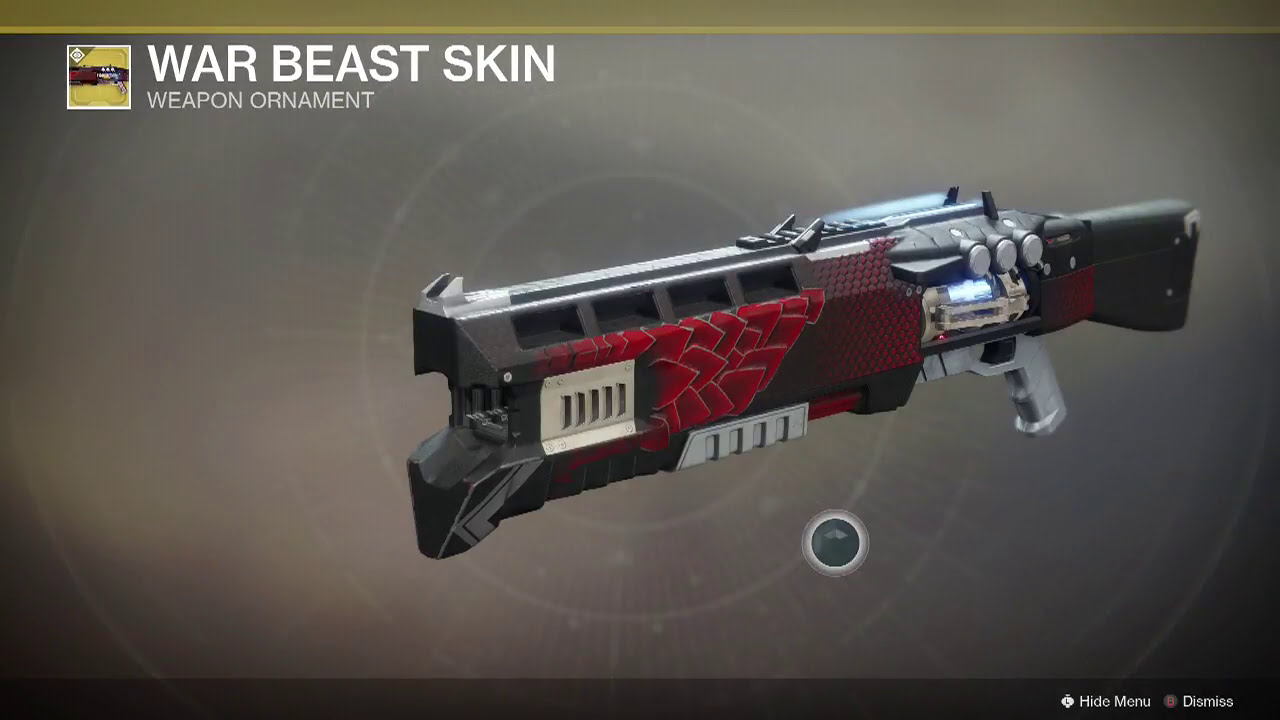The image is a detailed screenshot from the game Destiny, showcasing a futuristic shotgun with a distinctive War Beast Skin weapon ornament. The gun features a combination of silver and red colors with black accents, and has a scaly feather-like pattern on its barrel. A glowing section suggests it might be a high-tech laser or energy weapon. The gun includes a rifle butt, a handle with a trigger, and several knobs, emphasizing its advanced design. In the upper left corner, white text reads, "War Beast Skin," followed by "Weapon Ornament" in smaller letters. The background has an alchemy table design with circles and lines converging at the gun. In the bottom right, two buttons labeled "Hide Menu" and "Dismiss" are visible, indicating this is an in-game interface.